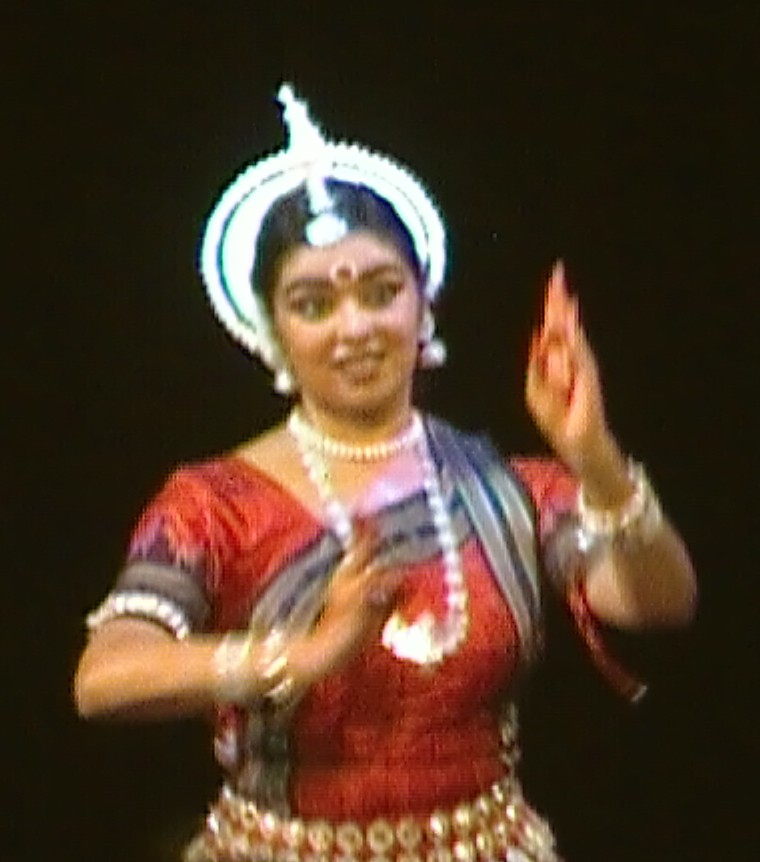The photograph is a grainy, digitized image of an Indian woman dancing against a solid black background. Captured from the waist up, the woman is adorned in a traditional, ornate red sari accentuated by a gold belt. Draped over her is a silver scarf that complements her attire. She wears an intricate white beaded headdress that frames her pulled-back black hair, and her ears are adorned with large, white dangling earrings. Her forehead features a red gem outlined in gold, centrally placed between her eyebrows. Her eyes are accentuated with black paint, and she boasts a dual-tiered necklace of pearls – a short one tight to her neck and a longer strand that cascades down her chest. Her arms are decorated with multiple bracelets, and her hands are depicted in mid-movement, one held up and the other across her chest, with fingers pointing gracefully as part of her dance. The photograph has a sense of performance, with her blurred hands conveying the dynamism of her traditional dance.